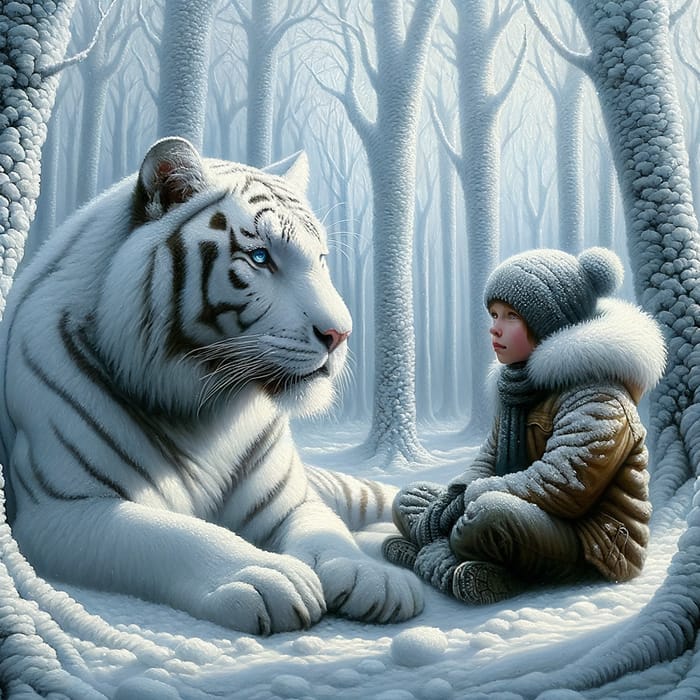In this meticulously detailed, high-resolution vertical image, likely a product of either advanced digital illustration or AI generation, a serene winter scene unfolds. At the heart of the image, a small child, dressed in a heavy brown parka with a furry hood, a knitted cap, and gloves, sits cross-legged in the snow. The child's calm demeanor exudes a surprising elegance and tranquility, despite the unusual presence of a majestic white tiger with striking blue eyes.

The tiger, adorned with brown stripes, rests gracefully on the left side of the image, seemingly lost in the distance, oblivious to the child at its side. Snow gently dusts both the child and the tiger, contributing to the serene winter atmosphere. In the background, barren trees, their bark laden with snow, frame this unlikely duo. The snow appears almost surreal, with small orbs adding a touch of the fantastical to the scene, further suggesting the image’s digitally altered nature. Despite the setting's fantastical elements, the composition captures an enchanting moment of quiet companionship between child and beast amidst a snowy forest.